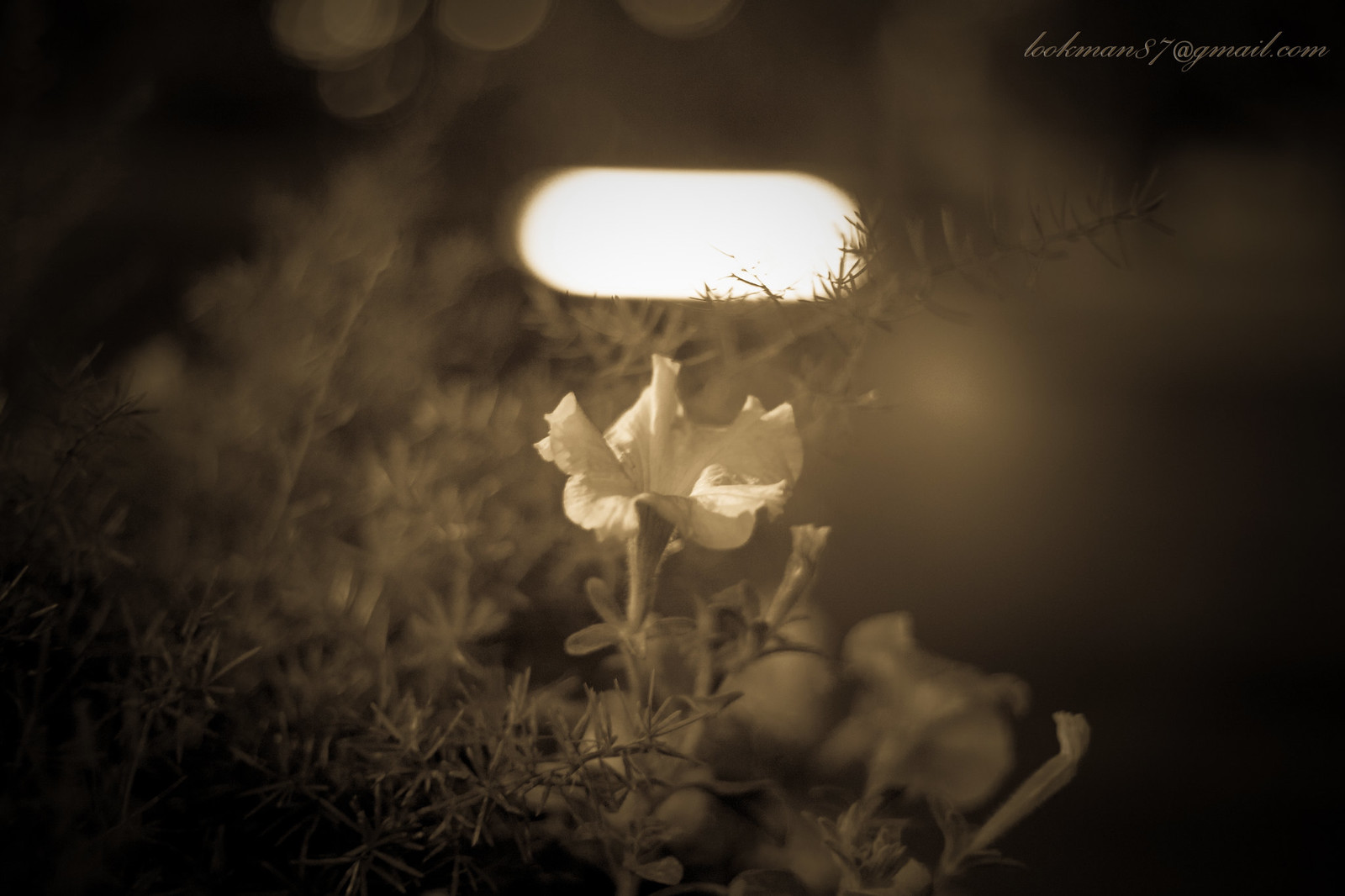This black and white photograph, with sepia tones, captures a delicate, white petunia bloom as its central focus. The petunia, characterized by its flowy petals, stands prominently amidst needle-like green foliage that extends from the bottom to the top of the image. The surrounding environment includes various leaves, stems, and branches, suggesting it may be part of a bush or vine. To the right of the main flower, some smaller, half-closed petunia blooms are visible. The background becomes increasingly indistinct and dark towards the edges, creating a soft blur that enhances the contrast with the illuminated flower. A bright, oblong, horizontal light source, resembling a fluorescent or neon light, shines from above the flower, casting a gentle glow that highlights the central bloom. The top right corner of the image bears the signature "Beckman87@gmail.com," possibly the photographer's contact or business information. The overall composition draws attention to the ethereal beauty of the petunia amidst its natural surroundings.